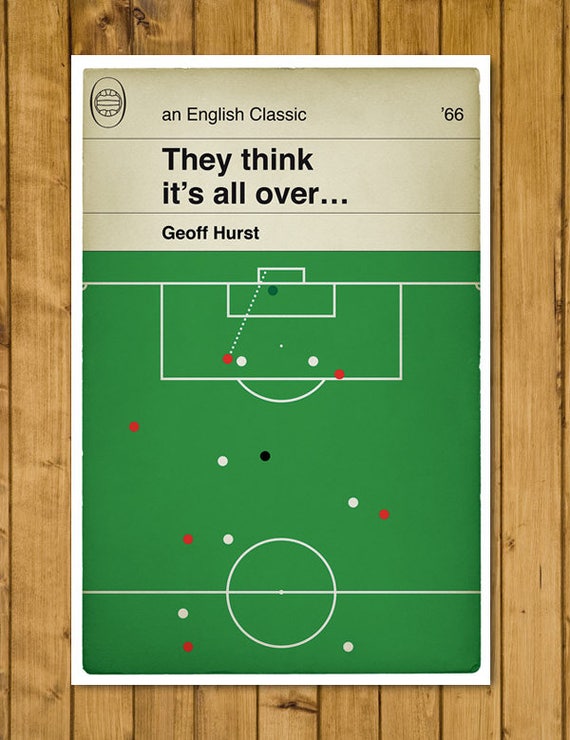This detailed poster, displayed against a wood-paneled wall, features the title "They Think It's All Over" by Geoff Hurst, with "An English Classic" inscribed at the top in black writing against a brownish-white background. The top right corner includes the numbers "'66," likely referencing the year 1966. The upper left-hand corner of the poster features an oval logo that may depict a soccer ball, characterized by a non-traditional design. Below, the poster transitions into a green soccer field diagram, marked by a thin white border. The field layout shows a white line and a center circle, goal boxes, and penalty arcs. Yellow and white dots scattered across the field represent the teams' players, with a black dot central to the layout. The red team is indicated with six red dots, and the white team with seven white dots, emphasizing the strategic player positions. This diagram captures a classic English soccer play in detailed visual form.